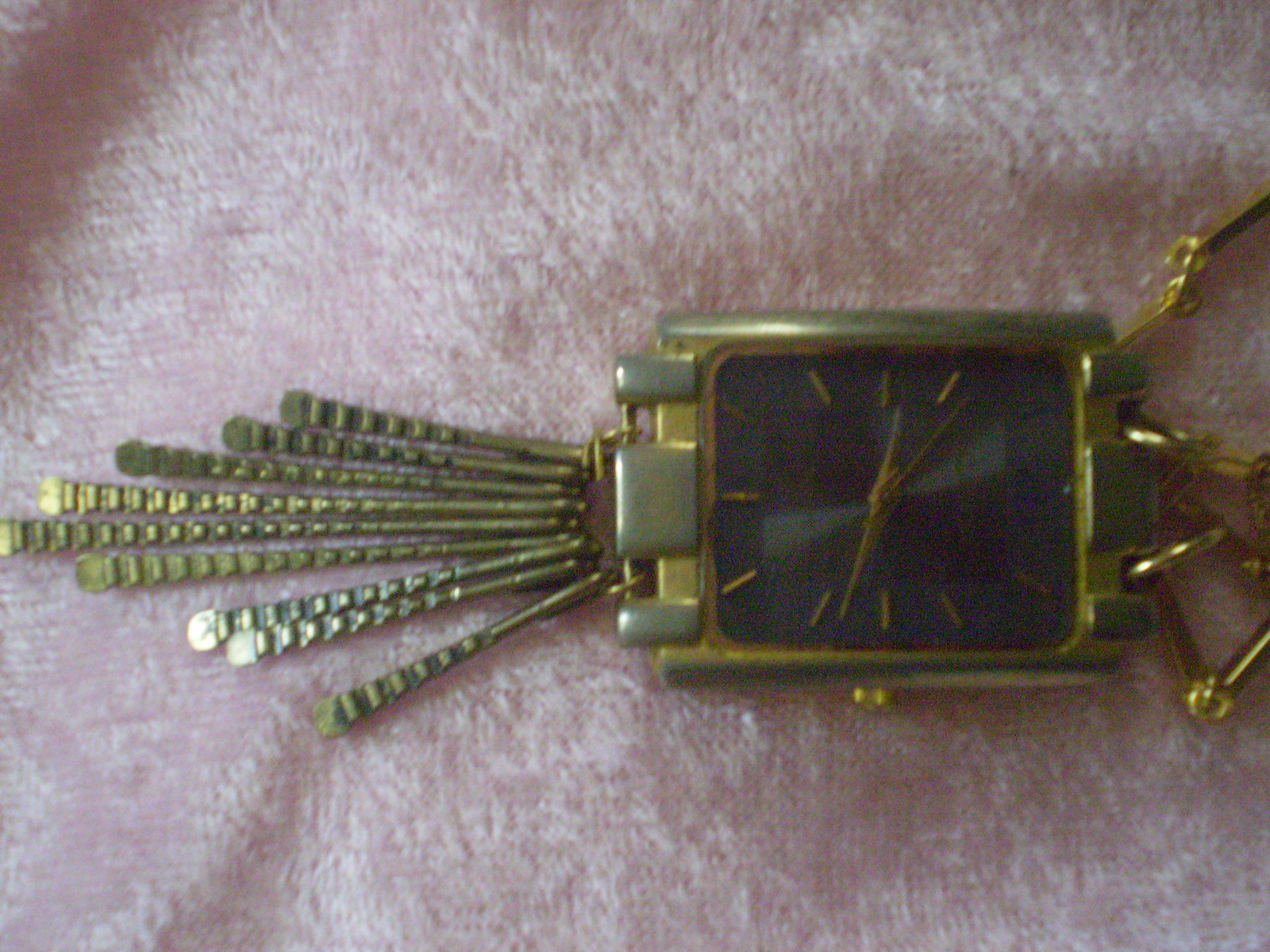A close-up photograph showcases an unconventional watch design, likely part of a necklace. The watch rests on a pastel pink, fuzzy fabric, creating a soft, delicate backdrop. The watch face appears to be a dark green, though the dim lighting in the image makes the exact color difficult to discern. The watch hands and hour markers are gold, standing out against the watch face. The minimalist design features only these gold lines without any numbers. Surrounding the watch face is a brass frame, which may have greenish details—though it's unclear if this hue is due to natural patina or lighting. Overall, the intricate details of the watch are set off by the cozy, textured fabric beneath it.